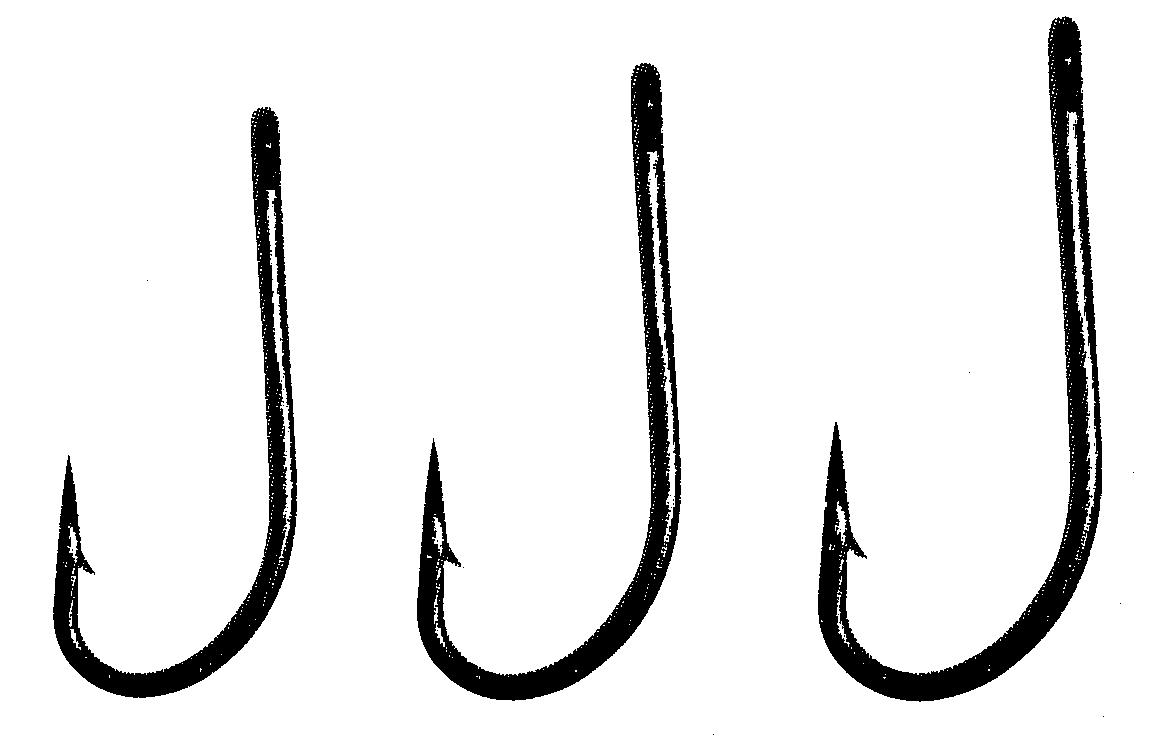This image features a black and white illustration of three fish hooks, resembling a pencil or charcoal drawing on a white background. Each hook is positioned side by side, creating a sequence from left to right. The smallest hook is on the left, identifiable by its very sharp and fine point, along with a little tail after the edge possibly featuring a dot for nailing. The middle hook is slightly larger, mirroring the design of the first with its black body accented by white along the side and by the hook. The largest hook, on the right, has more pronounced white detailing. All hooks share a distinct J-shaped formation, with openings at the top for threading a line, and each culminates in a very sharp, pointy end.